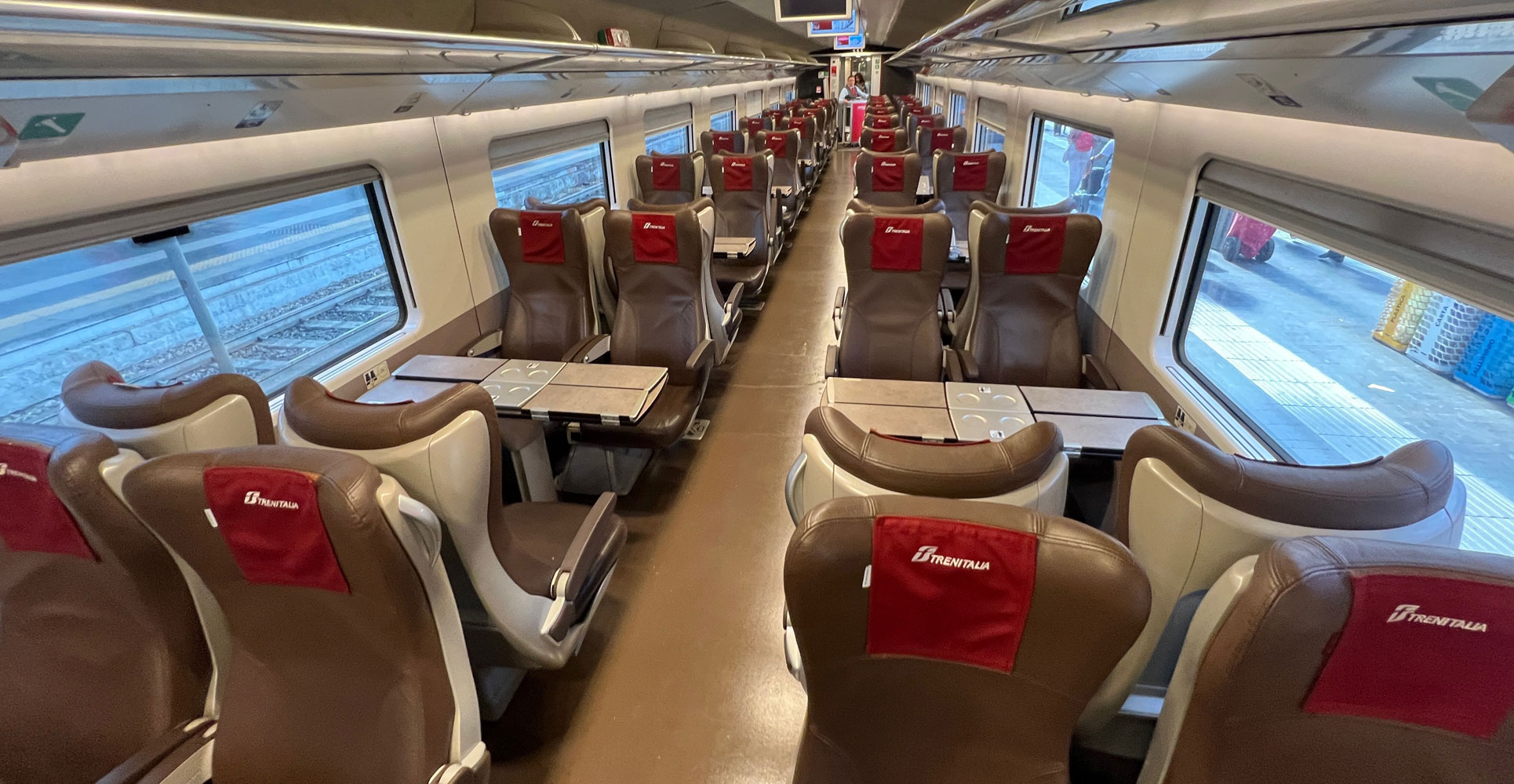This image captures the interior of a train carriage, looking down a wide aisle lined with rows of seating. The seats are upholstered in a brown, leather-like material and are arranged in facing pairs around compact tables. Red cloth headrest covers, inscribed with "TREN ITALIA," are affixed to the top of each seat. The spacious interior features large windows that offer views of train tracks on one side and a platform on the other. The floor is a matching brown color, complementing the overall beige and cream color scheme of the train's interior. Mounted on the ceiling are screens spaced along the middle axis of the carriage. A person standing at the far end of the aisle appears to be handling a cart, possibly for refreshments, ready to service the empty seats.